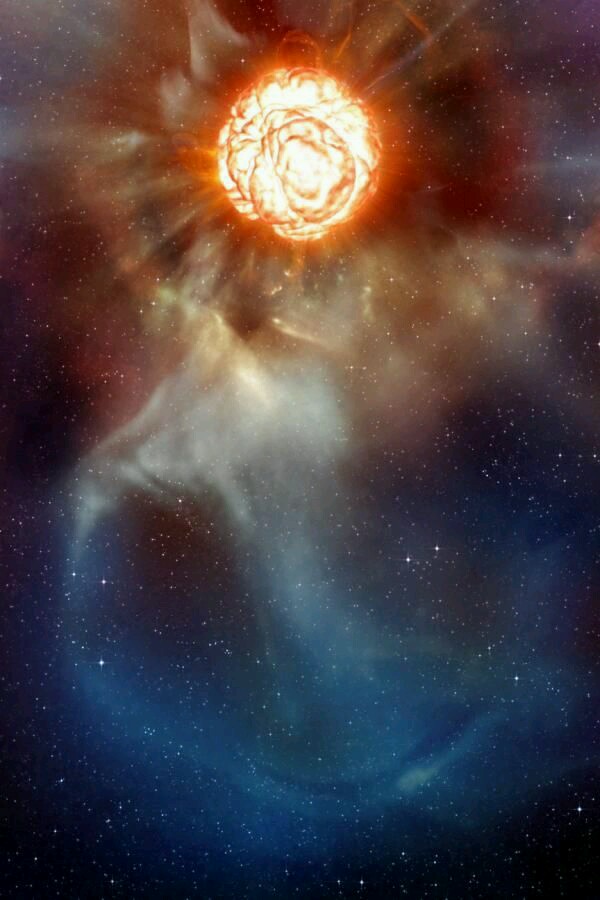This is a detailed artist's rendering of a dramatic explosion in outer space. Central to the image is a round fireball predominantly colored bright red and orange, reminiscent of the sun, situated near the top center. The explosion radiates outward in a striking display of icospheric symmetry, revealing fiery debris and clouds in an axisymmetric pattern. The explosion's core gleams white, surrounded by a dynamic mix of colors including blues, purples, and reds, transitioning to blues and cloudy formations at the bottom. All around, the vast starry backdrop features countless white stars of varying sizes, alongside scattered hues of black, light green, yellow, and white, giving the scene a mesmerizing aurora borealis-like effect.